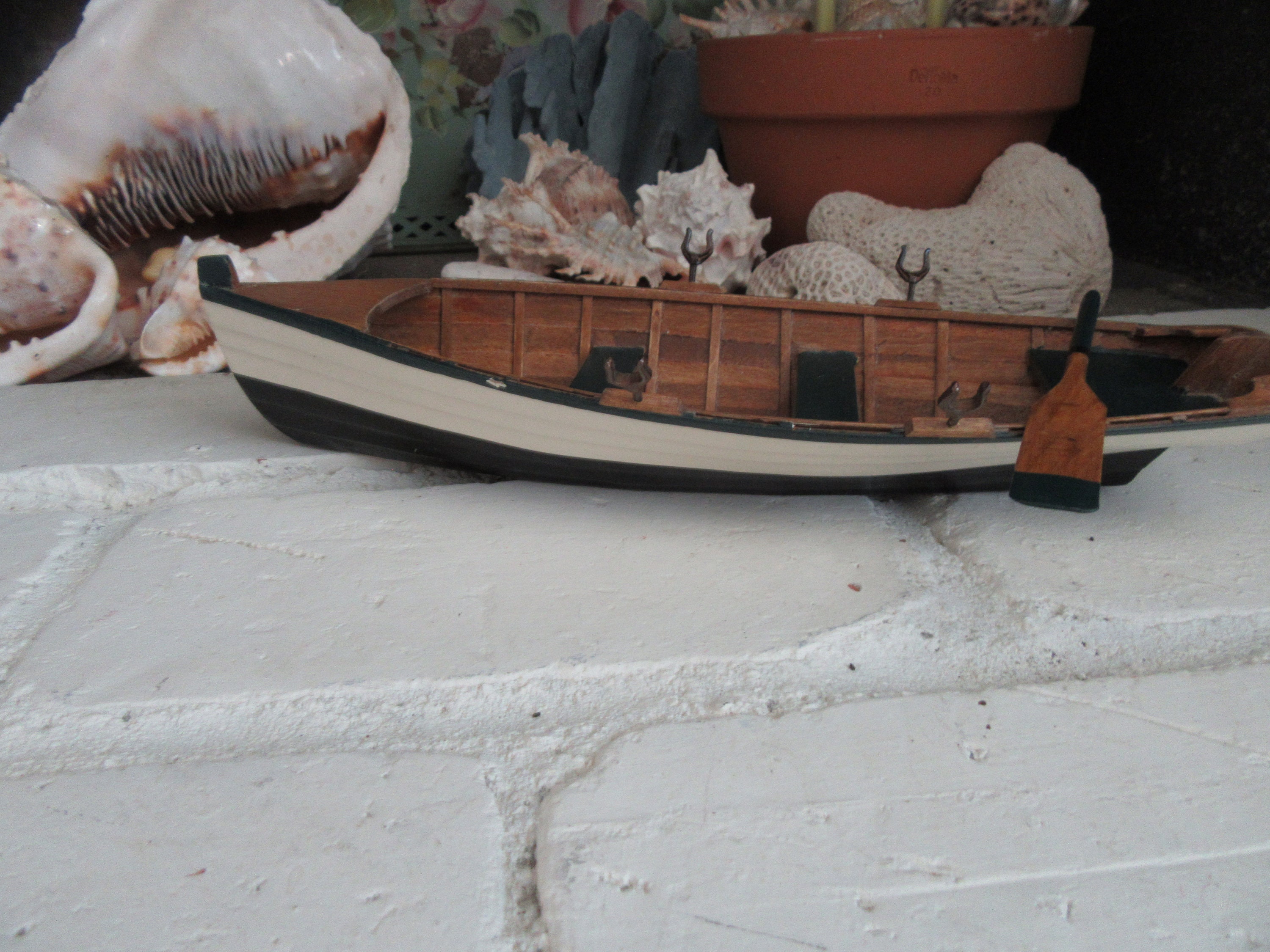The image features an artfully decorated white brick mantel adorned with various nautical-themed items. Central to the display is a meticulously carved wooden model of a canoe, approximately 12 inches long. The canoe boasts a brown interior and a thin black stripe along its top edge, complemented by a white banner on its side. The bottom portion of the canoe is also black. Leaning against the right side of the canoe is a small wooden paddle, also brown with a black handle and black-bordered bottom. Above and around the canoe, white seashells, including an extremely large conch shell with a darker brown interior on the left, are scattered, creating an arrangement that surrounds the base of a terracotta clay pot. The pot is placed behind the canoe and seashells, adding a rustic touch to the nautical display. This carefully curated scene is set against the clean, white stones of the mantel, with white grout accentuating the structure. The contrast between the dark and muted colors of the decorative items and the white background creates a visually striking and cohesive maritime display.